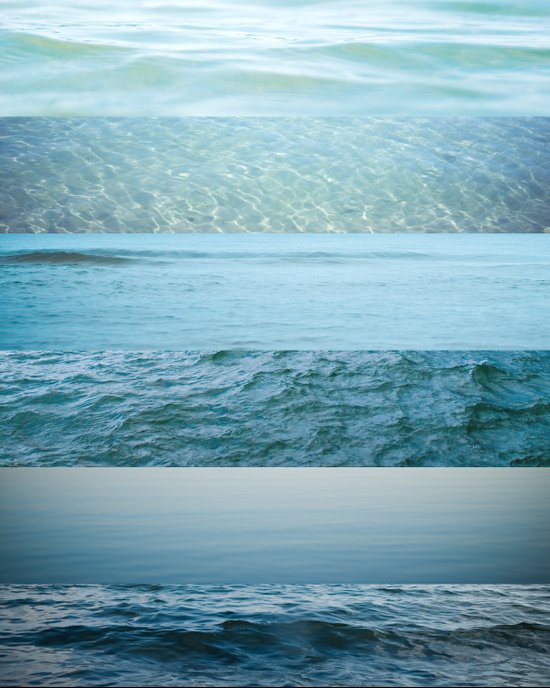This image is a composite of several different photographs of water, arranged in columned rows, each showcasing varying states and shades of the ocean. The top section displays light blue-green water with soft, gentle waves, evoking a restful feel. Below that, another photograph captures the sunlight dancing in the water, creating soft ripples in a slightly darker blue hue. The third image features a medium blue ocean vista with dark, distant waves, giving a clear, calm impression. Beneath this, a darker, almost gray scene shows rougher, choppier water, reminiscent of rocks or pebbles beneath the surface. The fifth section presents still, glossy water in a light blue shade, with scattered white ripples signifying gentle movement. The final image is markedly darker, with an almost gray-black hue and prominent, rippling waves, creating an impression of angry, turbulent waters. Altogether, the hues range from light teal to dark blue-gray, highlighting the diverse and dynamic nature of large bodies of water, such as oceans or lakes.